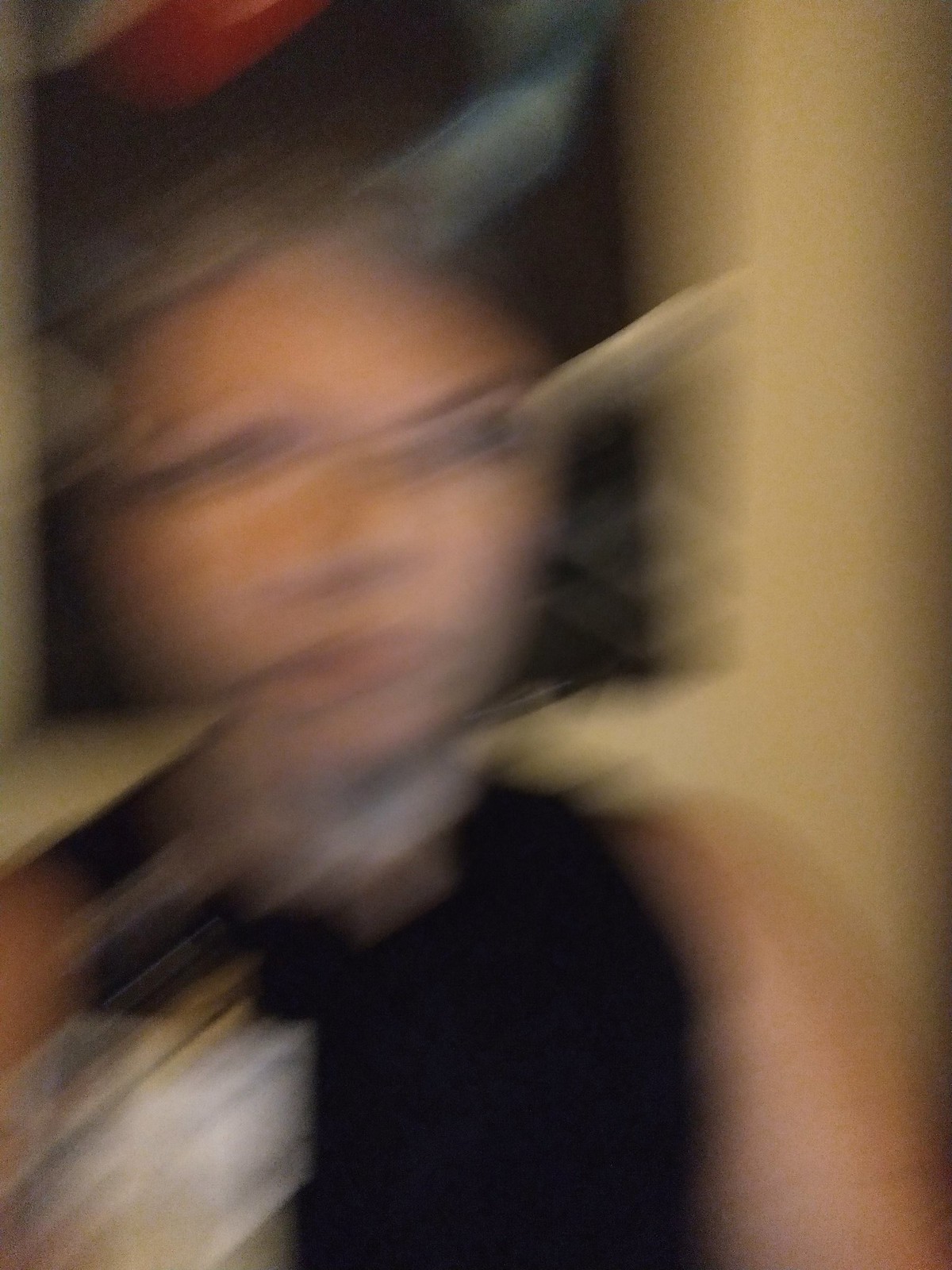This image features a double-exposed, somewhat blurry portrait of a Caucasian woman with a heart-shaped face. Her serious expression is accentuated by dark eyebrows and dark blonde hair, as she gazes slightly toward the right-hand side of the frame. The lower part of the image fades into a dark, indeterminate space that suggests she may be wearing dark clothing. To the right of her face, a fleshy structure, possibly a thumb, appears to touch or hold her chin. The right side of the image contains hazy, translucent, squarish shapes that may resemble a window frame and other indistinct structures. These elements are diagonally oriented, leading into the picture from the bottom left corner. Additionally, several blurry, streak-like lines traverse the image diagonally, varying in shades of gray, clear, and beige, adding to the ethereal and fragmented nature of the photo.